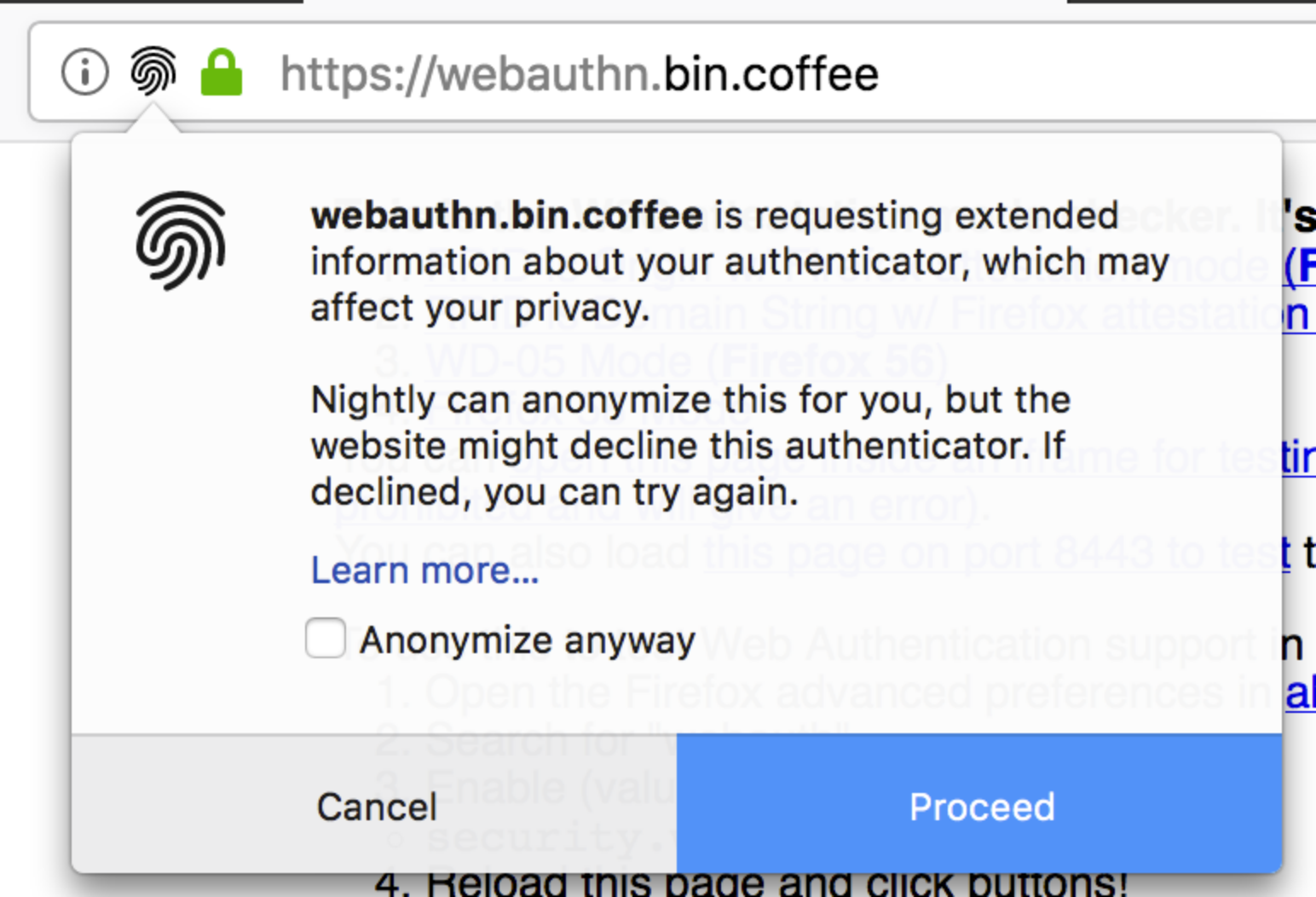This screen grab captures a webpage with a colorful interface consisting of black, green, white, and blue elements. At the top, a white navigation bar contains the web address "https://web.authn.bin.coffee," accompanied by a green padlock icon, a black swirly fingerprint icon, and a gray circle with an eye icon. 

A white pop-up window is prominently displayed, featuring a warning message in black text: "web.authn.bin.coffee is requesting extended information about your authenticator, which may affect your privacy. Nightly can anonymize this for you, but the website might decline this authenticator. If declined, you can try again." Below the message, a blue link labeled "Learn more" is visible, followed by an unchecked white box labeled "anonymize anyway." At the bottom of the pop-up, there are two buttons: a gray "Cancel" button and a blue "Proceed" button.

Behind the pop-up, the webpage background is white with interspersed black and blue text. The visible text includes instructions that read, "Reload this page and click buttons," and the number "4" is discernible at the bottom of the image. The overall image quality is excellent and clear.